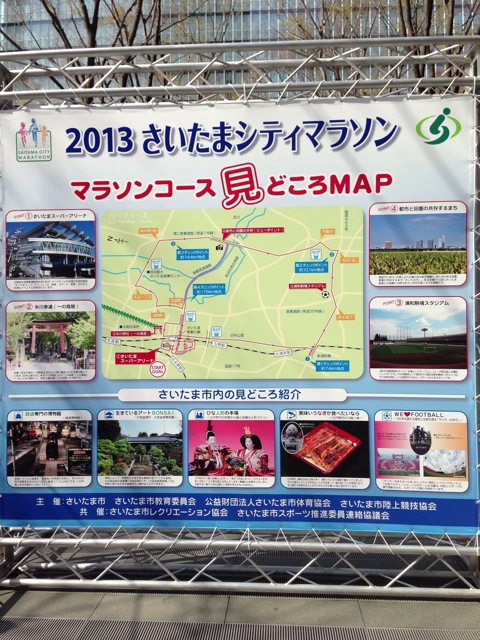In this image, a large outdoor poster in Japan is displayed, held up by metal bars at both the top and bottom, with white ropes securing it. The poster prominently features the year "2013" in blue numbers, followed by a series of Japanese characters in red font. Adjacent to this, the word "map" is displayed in English. Central to the poster is a detailed map with various callouts pointing to different tourist attractions, shown through numbered and colored tabs. Surrounding the map on the left, right, and bottom are numerous photographs depicting these attractions, including buildings, gardens, and people in traditional Japanese attire. At the bottom of the poster, there's a dark blue strip containing additional Japanese writing in white.